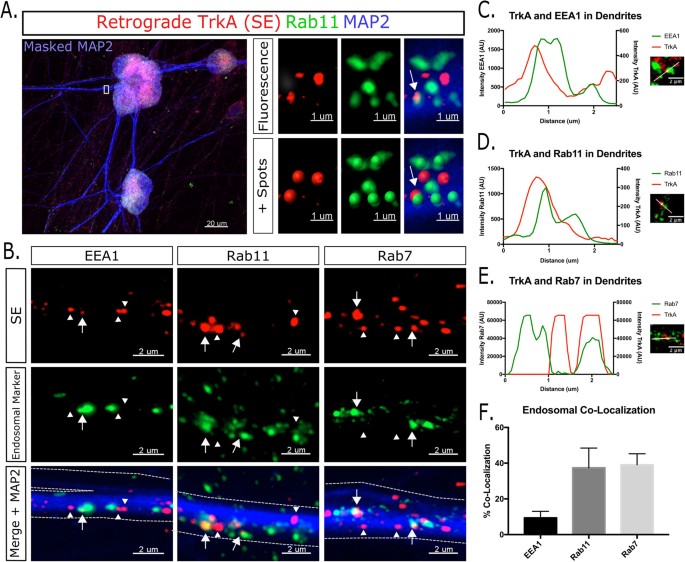This detailed scientific diagram, titled "Retrograde TRKASERAB11MAP2," is segmented into sections A through F, each containing a variety of visual data representations. 

Section A features intricate designs of molecules and spots marked by fluorescence, showcasing colorful lights typical of microscope imaging. This section presents diagrams labeled with EEA1, RAB11, and RAB7, highlighted by red and green dots and interconnected by blue line waves.

Section B displays six smaller images, denoted as MERGE plus MAP2, which also feature the endosomal markers SE, EEA1, RAB11, and RAB7. These images consist of glowing, hazy dots in multiple colors, laid out on a black background.

Section C contains a detailed line graph labeled "TRKA and EE1 in dendrites," illustrating complex data points and trends.

Similarly, Section D presents another line graph labeled "TRKA and RAB11 in dendrites," whereas Section E shows a line graph for "TRKA and RAB7 in dendrites."

Finally, Section F concludes with a bar chart labeled "endosomal colocalization," comparing various data points related to the colocalization of endosomal markers.

This diagram collectively represents a sophisticated array of scientific data on endosomal markers and their fluorescence under a microscope, offering a multifaceted view of molecular activity.